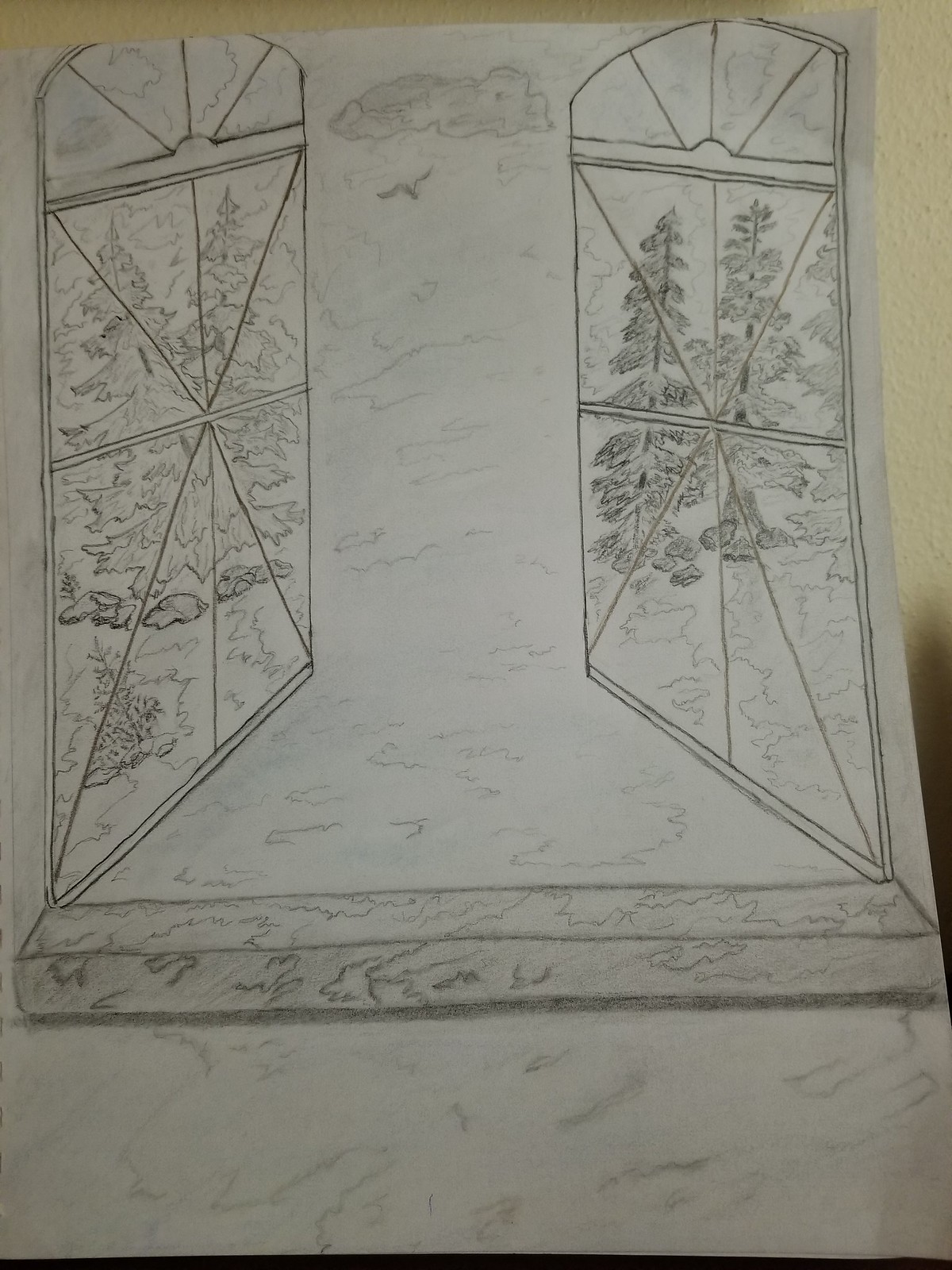The image is a detailed pencil sketch on a plain white piece of paper, depicting an open window framed by an archway-shaped extension at the top, beyond a horizontal bar. The window's intricate bars extend in multiple directions—left, right, top, bottom, and diagonally—creating a pattern across the panes. The windowsill and wall below are sketched to resemble marble, with subtle, swirly gray lines adding texture. Outside the window, a serene field is visible, flanked by trees on both the left and right sides. A tiny bird is captured mid-flight beneath a solitary, simple cloud in the sky. The panes of the window could be either stained glass or clear, adding an element of visual ambiguity as the trees appear both on the glass and beyond it.